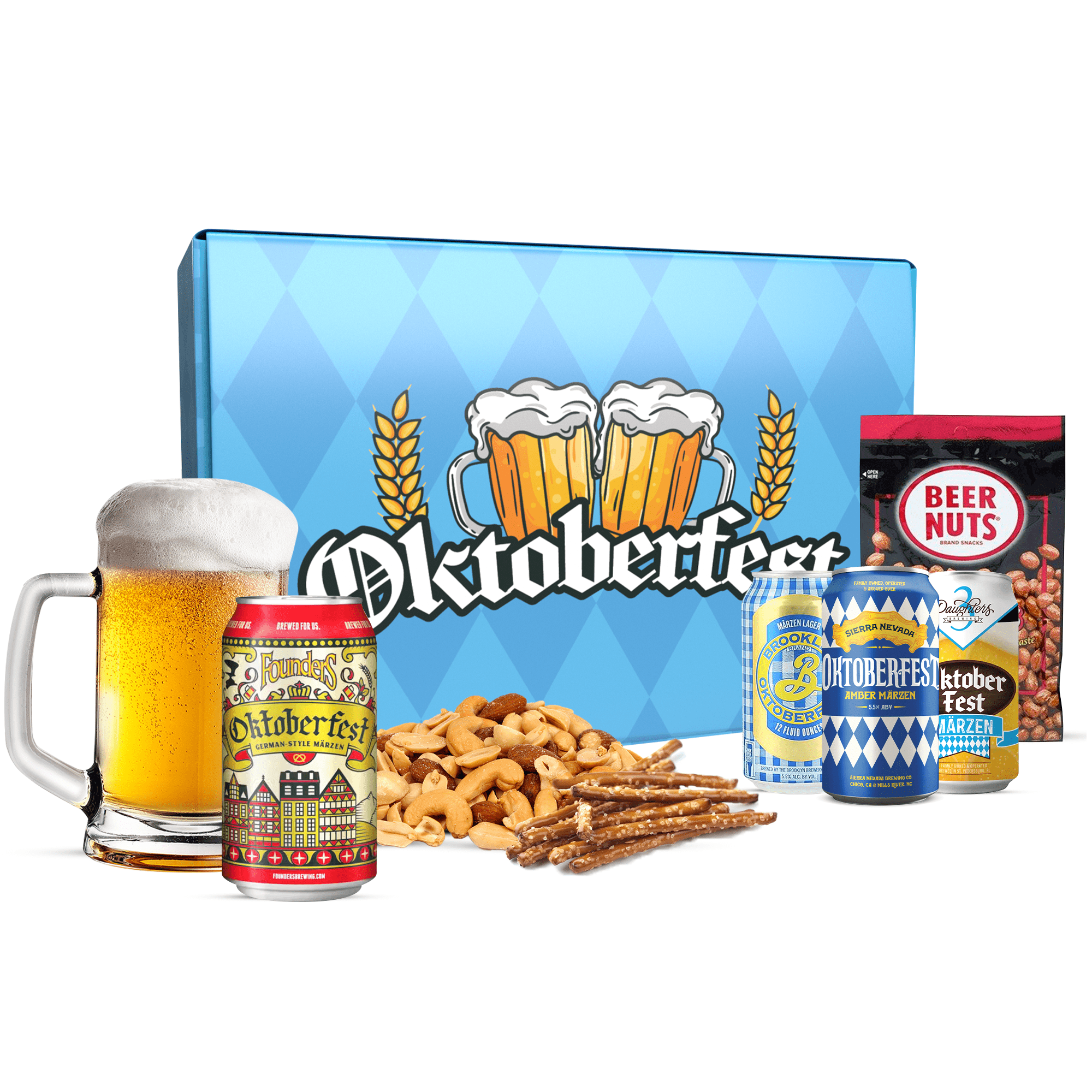The image features a vibrant Oktoberfest display set against a white background, evoking the celebratory spirit of the renowned festival. Central to the scene are multiple beer mugs filled with frothy, amber beer. Prominently displayed is a stein showcasing the Oktoberfest logo in yellow. Among the assortment, there are several cans of Oktoberfest-branded beer, adorned with festive colors and designs depicting typical German architecture. One notable can, placed next to the stein, features red and yellow hues with a depiction of German buildings. Other cans, predominantly in blue and white, also bear the Oktoberfest branding, including one labeled "Brooklyn Oktoberfest." Surrounding the beers is an array of snacks: mixed nuts including cashews, almonds, and peanuts, along with brown pretzel sticks, emphasizing the traditional accompaniments of the festival. A pack of beer nuts, distinguishable by its black and red packaging, is visible, boasting a clear window that showcases the nuts inside and branded in red letters. In the background, there is a decorative box featuring an Oktoberfest theme with blue diamond patterns and an illustration of two clinking beer steins.